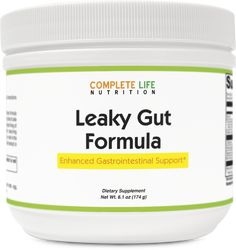An image of a white canister prominently displays a product titled "Leaky Gut Formula" on its white label with bold black lettering. The brand name, "Complete Life Nutrition," is written above, with "Complete" in red, "Life" in green, and "Nutrition" in black, all in capital letters. The label is bordered in green and features a gold-highlighted box on the front, proclaiming "Enhanced Gastrointestinal Support." The sides of the canister contain additional product information, though it is not fully visible in the image.